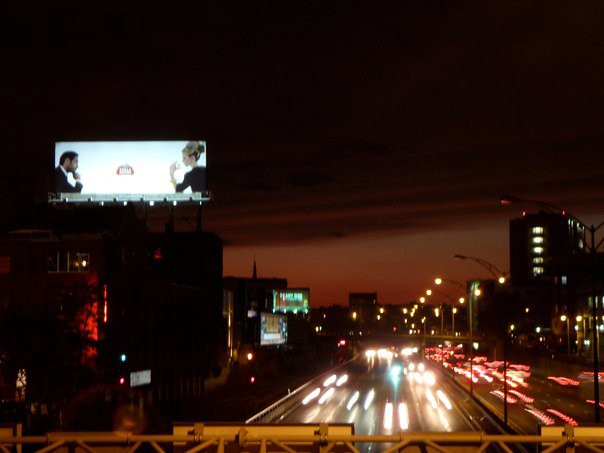Nighttime Cityscape with Traffic Light Trails

This photograph captures a bustling cityscape at night, showcasing the mesmerizing effect of light trails created by moving vehicles. The scene is dominated by two sections of the freeway, one heading towards the camera in the middle of the photograph and the other receding from the viewer on the right side. The light from the cars creates stretched streaks, giving a sense of motion and energy.

To the right, in the distance, a tall building stands prominent amongst a cluster of other buildings lining the freeway. On the far left of the image, a brightly illuminated billboard catches the eye. The billboard features a man in a suit with a beard, thoughtfully resting his hand on his chin, and a woman in a women's suit with her hair secured in a claw clip, poised with her fists up as if ready to fight.

Further back in the center, another billboard is visible, adding to the urban setting. The backdrop of the city is shrouded in a muggy haze, giving the sunset an ethereal, muted glow and adding a layer of depth to the atmospheric evening scene. Various other buildings and billboards dot the landscape, contributing to the vibrant, energetic vibe of the city at night.